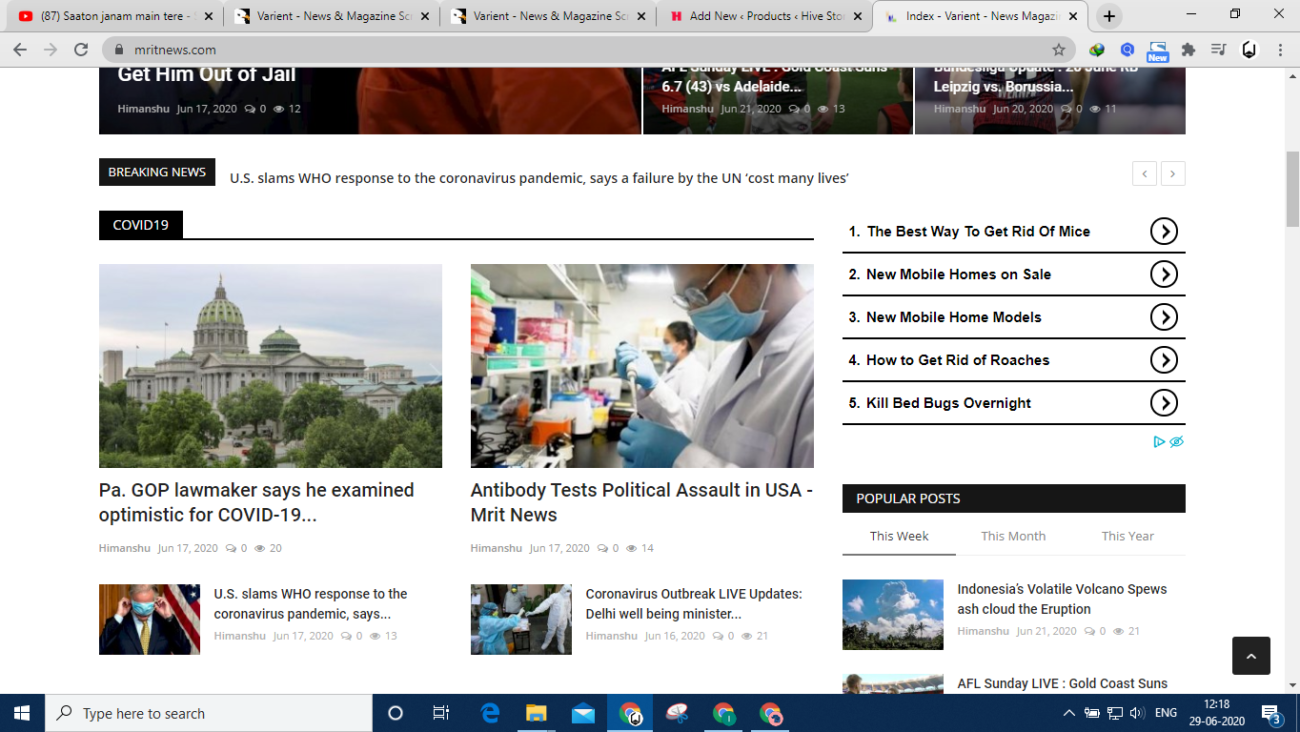This screenshot displays a section of the MRITnews.com website, featuring a dynamic layout with a variety of news articles and advertisements. In the header, it shows the website's logo "MRIT News" prominently. The main headline reads "Breaking News: U.S. slams WHO response to coronavirus pandemic, citing a failure by the U.N. that cost many lives." An accompanying image depicts a person donning a mask, reinforcing the article about the WHO's response to COVID-19.

The following section highlights another significant piece under the "COVID-19" category: "PAGOP lawmaker tests positive for COVID-19," paired with an image of a government building surrounded by trees. Below, there's a graphic of scientists working in a laboratory with a caption reading "Antibody test sparks political debate in U.S." 

Adjacent to these stories, a sidebar features a bulleted advertisement listing: "Best way to get rid of mice," "New mobile homes on sale," "New mobile home models," "How to get rid of roaches," and "Kill bedbugs overnight." Additionally, a section labeled "Popular Post This Week, This Month, This Year" is visible, with "This Month" highlighted, showing articles like "Indonesia's volatile volcano spews ash cloud," and "AFL Sunday live, Gold Coast Suns."

At the top of the screen, there's an indication of multiple open tabs in the web browser, suggesting a user engaged in browsing several sites simultaneously.